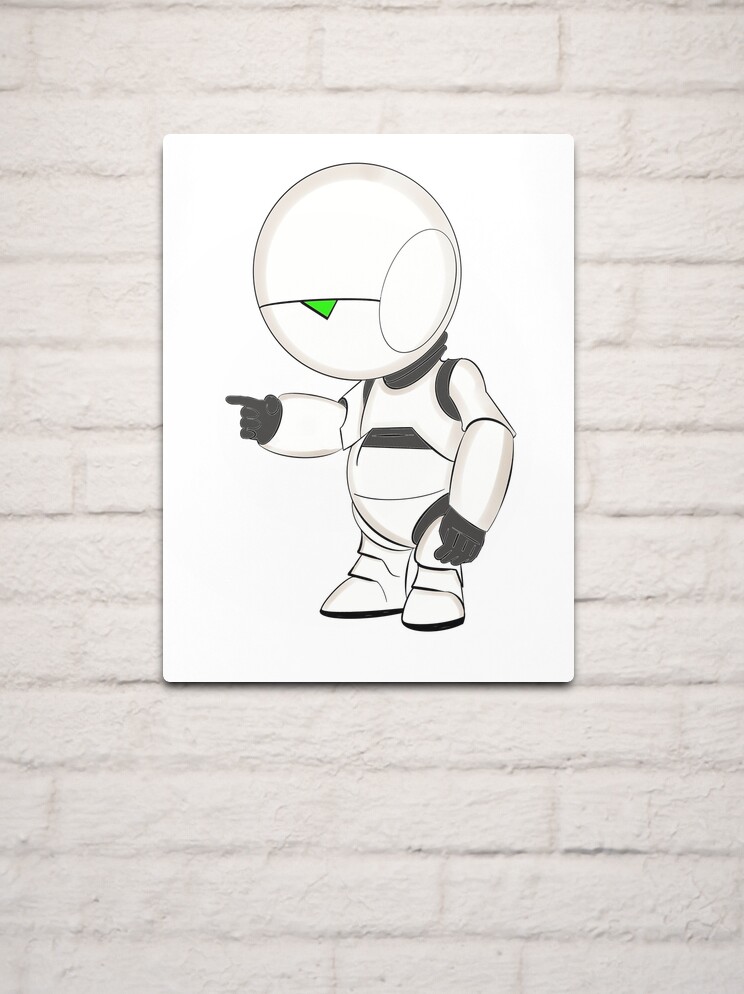The image showcases a meticulously detailed poster mounted on a white brick wall, featuring a character that highly resembles the robot from "The Hitchhiker's Guide to the Galaxy." The focal point of the art piece is a robot with a large, perfectly round head that could be seen as a helmet. This head features a distinct light green, upside-down triangular eye and is complemented by an oval-shaped ear delineated in black. The robot's body is predominantly white with intricate elements, such as a black neck and a horizontal line across the stomach, which also sports some black areas and ruffled texture for added detail. 

The robot is depicted in a side profile, with its black-gloved index finger pointed forward, imbuing a sense of action. Its feet are white with black soles, and the boots are sectioned for a more segmented look. A noteworthy detail above the chest is a black segment that appears to be connected to something, hinting at the robot's complexity. The overall composition is rendered on a white poster board, adding a polished, minimalist backdrop that emphasizes the robot's futuristic design and form.